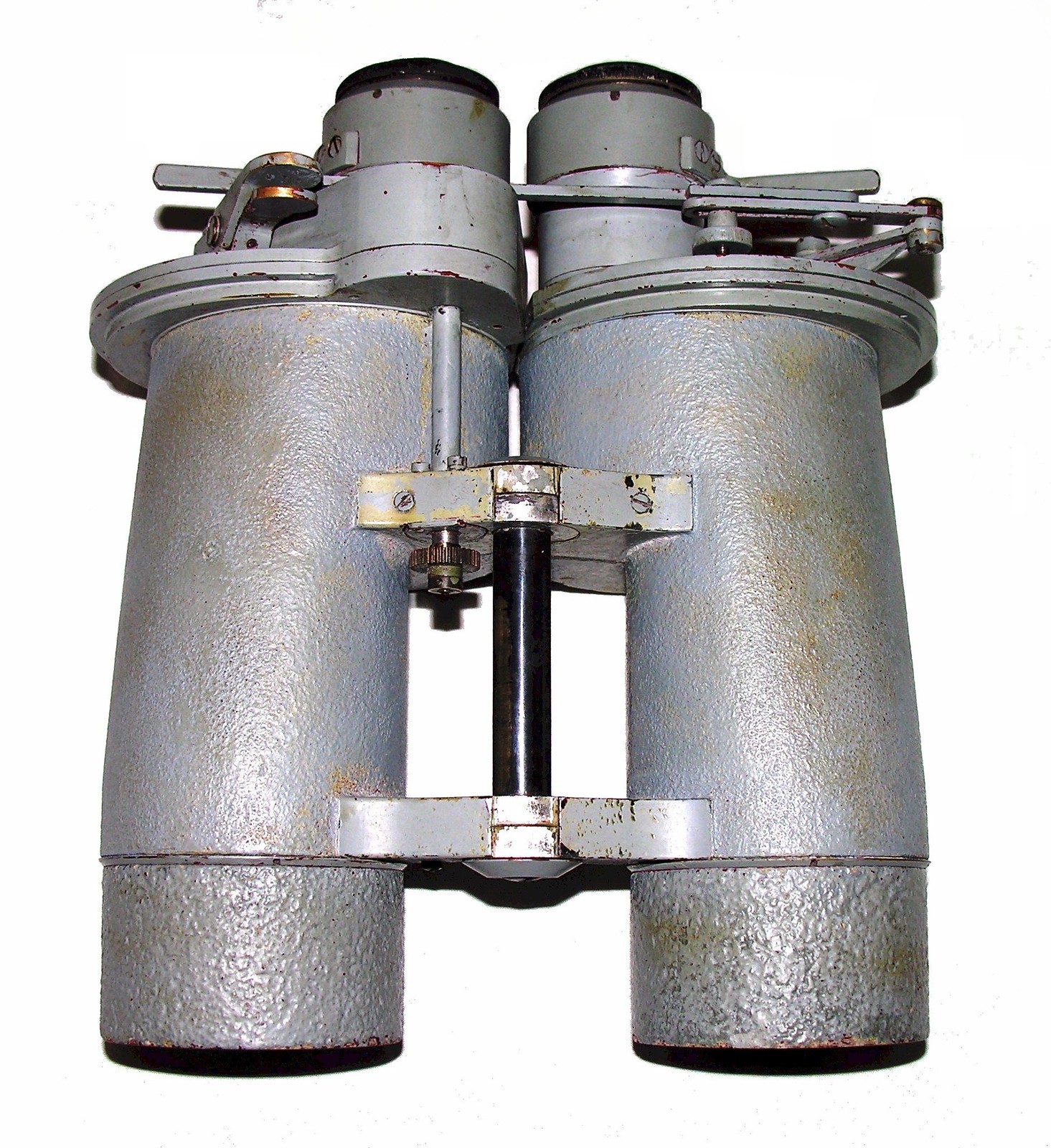The image features a top view of a pair of vintage binoculars set against a faint white background. These large binoculars have a worn, light gray metallic finish with patches of rust appearing as orange spots throughout the surface. The binoculars are composed of two long, rounded cylinders connected by a thick, light gray metal bar at the bottom center and a black bar at the back, which connects to a black metal plate. The surface is rough and bumpy. The eyepieces, which appear very worn, have black, possibly rubber borders that are deteriorating. There are metal adjustments and brackets for fitting the nose, and screws can be seen on the top part of the binoculars. The overall structure appears to be from around the 1960s or earlier, emphasizing its vintage and well-used nature.